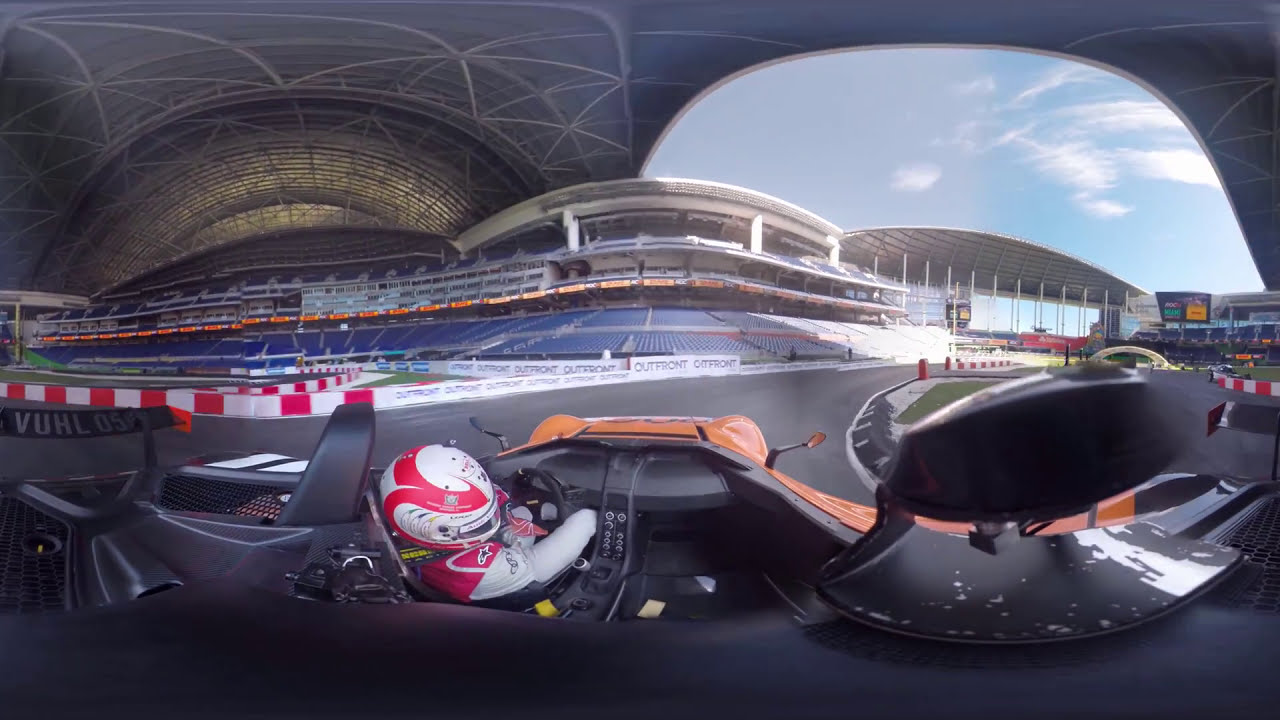A detailed, singular caption combining the provided descriptions could be:

"In this wide, horizontal 360° image, a race car driver is captured sitting in a vividly colored race car, which appears partially orange and yellow. The image exhibits noticeable distortion, warping the surroundings and the vehicle itself. The driver, wearing a distinct white and red helmet with an arrow-like design, and a matching white and red racing suit, is seated inside the car. Visible components include the gear shifter and the car's interior, suggesting a cockpit view.

In the background, the scene extends to a racetrack, bordered by empty blue grandstands, indicating a practice session rather than an ongoing race. The stadium is lit up, and reflective surfaces contribute to a doubling effect in some areas. To the right, a field and a partially visible sky with some clouds give the impression of a relatively clear day. Additionally, a white and red striped border is visible to the left center of the picture, and black text reading 'out front' is seen on the rail, hinting at a tunnel-like structure within the image. No other cars, drivers, or spectators are present, focusing the attention solely on the solitary driver and his vehicle."